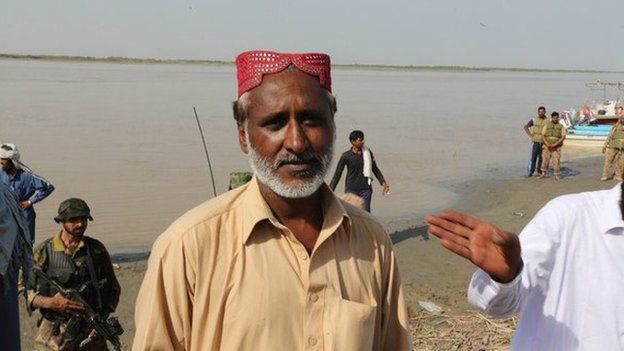In the foreground of the image, a Middle Eastern man with very dark brown skin is prominently featured, occupying about a third of the frame. He wears a distinctive red hat with a flat top and has a white-gray beard and mustache. His attire includes a tan, possibly mustard-colored, button-down shirt. He appears to be looking just to the right of the camera. The background reveals a beach area with dark, muddy water, indicative of a large murky lake or ocean. Behind the main subject, several other individuals are partially visible. To his right, there's a hand and part of the arm of a man wearing a white shirt. Below to the left, another man stands, identifiable by his darker shirt and a gunny-style hat, seemingly holding a rifle. Further back, a man in a white hat and blue shirt is also discernible. The image also includes military personnel; one soldier is fully equipped with military gear and holding a machine gun. Additionally, distant figures and potential boat silhouettes can be seen, suggesting the presence of military activity or possibly refugees set against a strip of green land in the background.